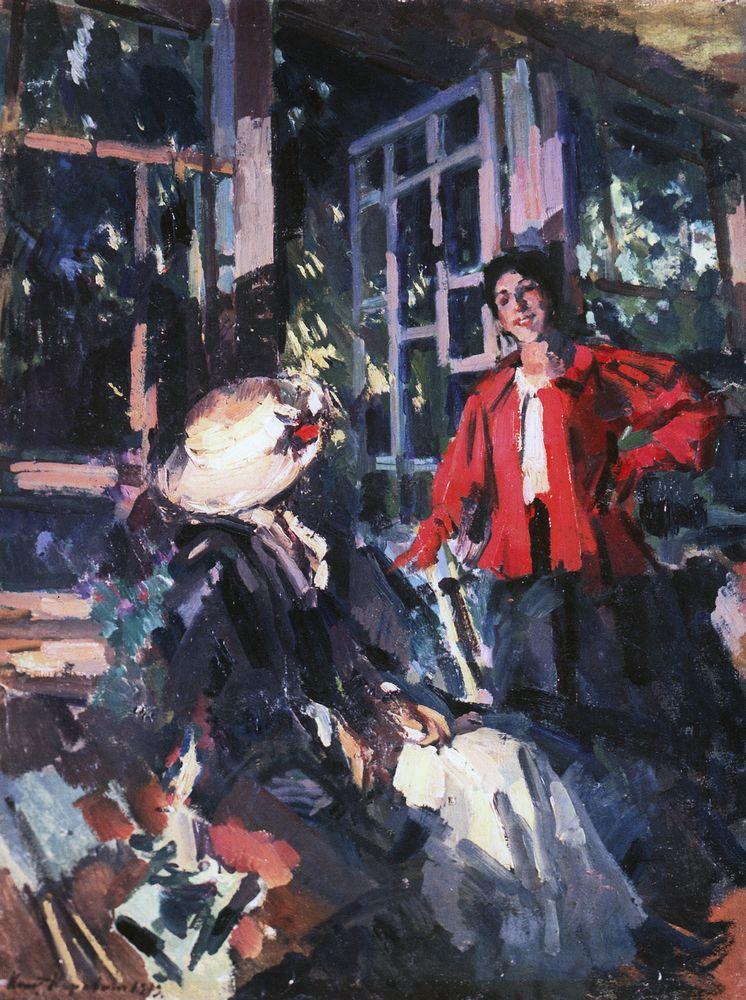The image depicts an oil painting in a post-Impressionist style featuring two women set against a vivid and complex background. The woman on the right is standing and facing the other figure, wearing a bright red jacket over a white shirt, with a hat that suggests she is female. She appears to be smiling warmly with her hand on her hip. The seated woman, positioned to the left, is dressed in cold blue hues and is looking up at the standing figure. The environment around them is somewhat ambiguous—possibly a greenhouse, café, or shed—accentuated by lush vegetation and an open door or window. The scene is bathed in a multitude of colors, including green, gray, blue, with various hints of red, yellow, black, brown, beige, orange, lavender, and tan, which blend to create a hard-to-define but richly colored tableau. The seated woman has a table next to her with indistinct items, further adding to the mystery and intrigue of the setting.